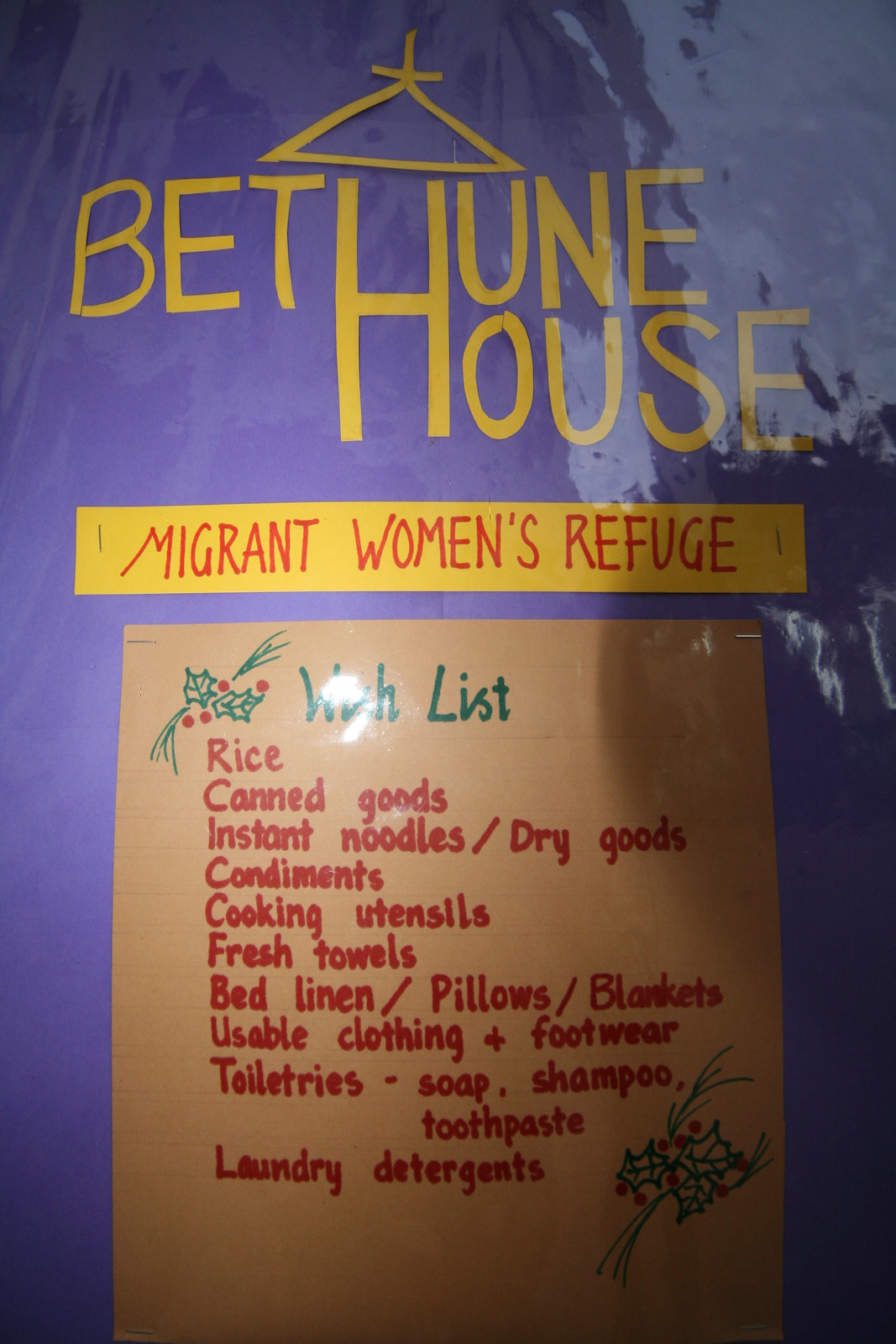The poster features a rich, light purple background and prominently displays the imagery and information for "Bethune House." The logo is stylized with a single large "H" serving both "Bethune" and "House," written in vibrant yellow letters. Above this logo, there is a triangular depiction resembling the roof of a house, possibly with a cross, which gives the structure an ecclesiastical feel. Below the logo, a bright yellow banner with red text reads: "Migrant Women's Refuge."

Underneath this banner, there is a Christmas-themed wish list adorned with pine needles and holly berries on a beige background. The heading "Wish List" is written in green, and the list outlines the items needed by Bethune House, written in red. The requested items include: rice, canned goods, instant noodles/dry goods, condiments, cooking utensils, fresh towels, bed linen/pillows/blankets, usable clothing and footwear, toiletries (such as soap, shampoo, toothpaste), and laundry detergents.